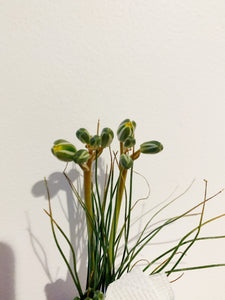The image features an indoor plant with a green stem, exhibiting a profusion of slender green leaves and numerous flower buds. The buds, numbering around ten, are primarily green with yellowish or orange accents at their tips, suggesting they are poised to bloom. These buds are perched on light brownish to orange-tipped stems, adding complexity to the plant's structure. The backdrop of the photograph is a plain, milky white surface, which accentuates the plant's vibrant greenery and the intricate shadows it casts. Positioned near the plant is a white cylindrical object, possibly a candle or a decorative item, contributing to the composition with its own shadow. The lighting, coming from the right side, enhances the depth and detail of the image, making the plant's various elements stand out against the clean background.